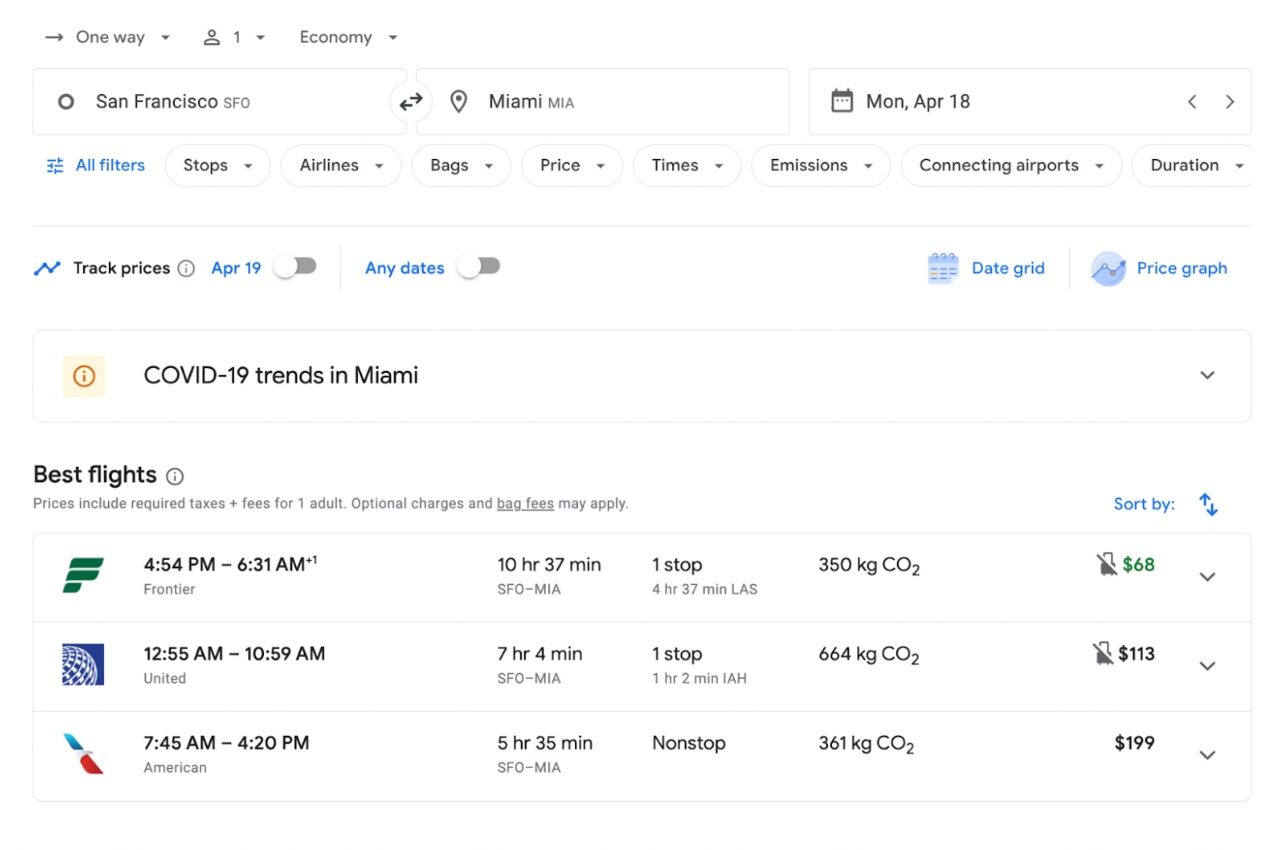This image showcases a flight booking screen designed for a website. In the top-left corner, there are options indicating a one-way trip for one person in economy class. Directly below, the flight details show a journey from San Francisco to Miami, set for Monday, April 18th.

The section below these details features nine filter categories: "All Filters" highlighted in blue, followed by "Stops," "Airlines," "Bags," "Price," "Times," "Emissions," "Connecting Airports," and "Duration" in black.

Further down, there is a "Track Prices" option dated April 19th, with the "Any Dates" toggle switched off. To the right, in blue, are two interface options: "Date Grid" and "Price Graph."

The subsequent portion includes a square icon denoting "COVID-19 trends in Miami."

The image also features a list of the best flight options:
1. **Frontier Airlines:** Departure at 4:54 p.m. and arrival at 6:31 a.m. with one stop. The price is displayed on the right at $68.
2. **United Airlines:** Departure at 12:55 a.m. and arrival at 10:59 a.m. with a duration of seven hours and four minutes. The price is $113.
3. **American Airlines:** Departure at 7:45 a.m. and arrival at 4:20 p.m. The flight duration is five hours and thirty-five minutes, priced at $199.

This detailed view ensures users can easily navigate their options and select the most suitable flight.